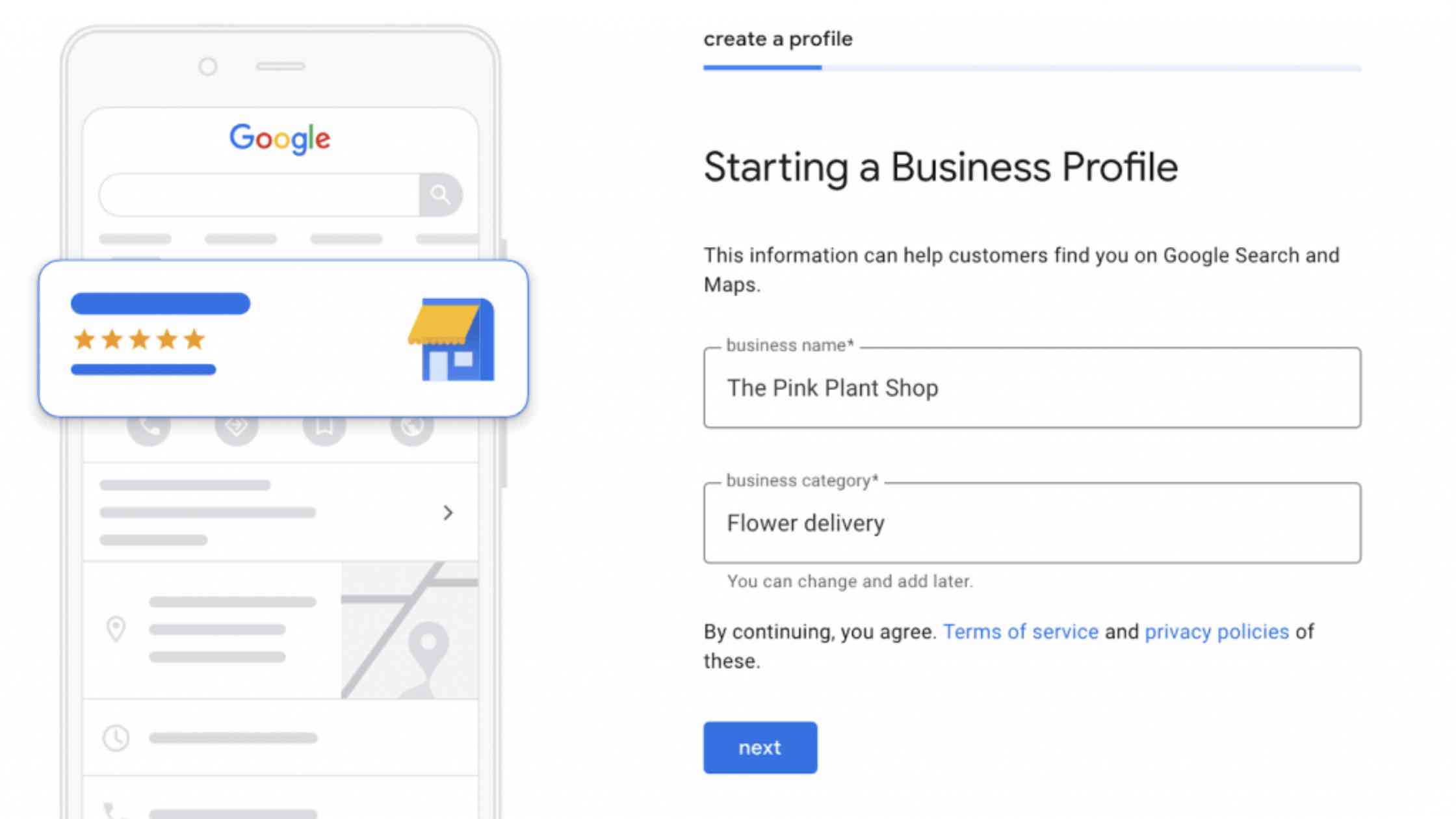In this image, we see the design elements of a profile creation page for a business. On the left side, there is an illustration of a mobile phone displaying five orange stars, indicating user reviews or ratings. The main section of the page shows the Google Search interface with a search field and a magnifying glass icon. Beneath this, there are various prompts and actions such as "Create a Profile" and "Start a Business Profile." The instructions inform the user that this process will help customers find their business on Google Search and Maps. The example business name provided is "The Pink Plant Shop - Flower Delivery." There is also a note stating that the business information can be updated later. At the bottom of the page, a disclaimer appears, mentioning that by continuing, the user agrees to the terms of service and privacy policies. A "Next" button is visible, indicating the progression to the next step.